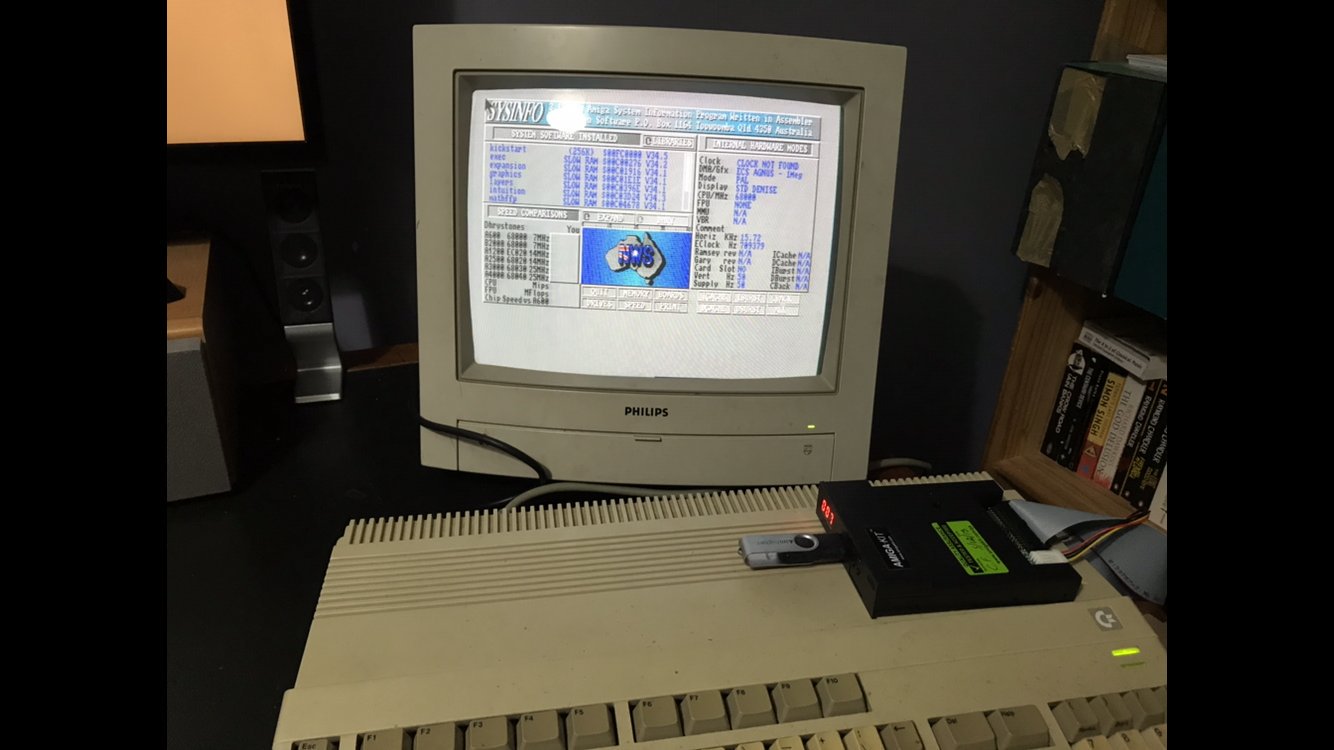This image captures a vintage Philips computer, likely from the mid to late 1980s, set up in a home office. The small, 8-inch square monitor features a prominent, plastic bevel and displays a SYS by NFO screen with what appears to be an older spreadsheet or chart program. Among the data on the screen, a map of Australia with blue markers can be seen, along with various numerical values. The keyboard, matching in vintage style, is large and bulky with light grey and dark grey keys. 

Below the screen, there's a disk drive situated on the front of the computer case. Sitting atop the keyboard, a black SD card reader with an inserted SD card is visible. The workspace includes additional equipment and furnishings, with the edge of a bookcase present on the right, and possible indications of a printer and desk lamp on the left. This setting is dimly lit, evoking a snapshot from a couple of decades ago.